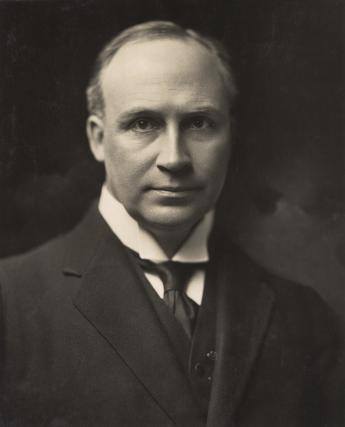In this black and white photograph, a middle-aged Caucasian man is portrayed facing directly towards the viewer. He has a prominent slight smirk and very short hair, which is slightly receded at the front and parted to his right. His attire is strikingly formal and old-fashioned, reminiscent of an Abraham Lincoln style, minus the hat. The man is dressed in a plain white collared shirt that resembles a tuxedo shirt, accompanied by a dark tie. Over his shirt, he wears a black vest and a matching dark suit jacket. The background of the photograph is predominantly black, gradually transitioning to a smoky, inconsistent gray near his shoulders, giving the appearance of ethereal clouds or smoke. This classic and somewhat staged setting suggests that the photograph might have been taken in a photo studio, adding to its timeless quality.